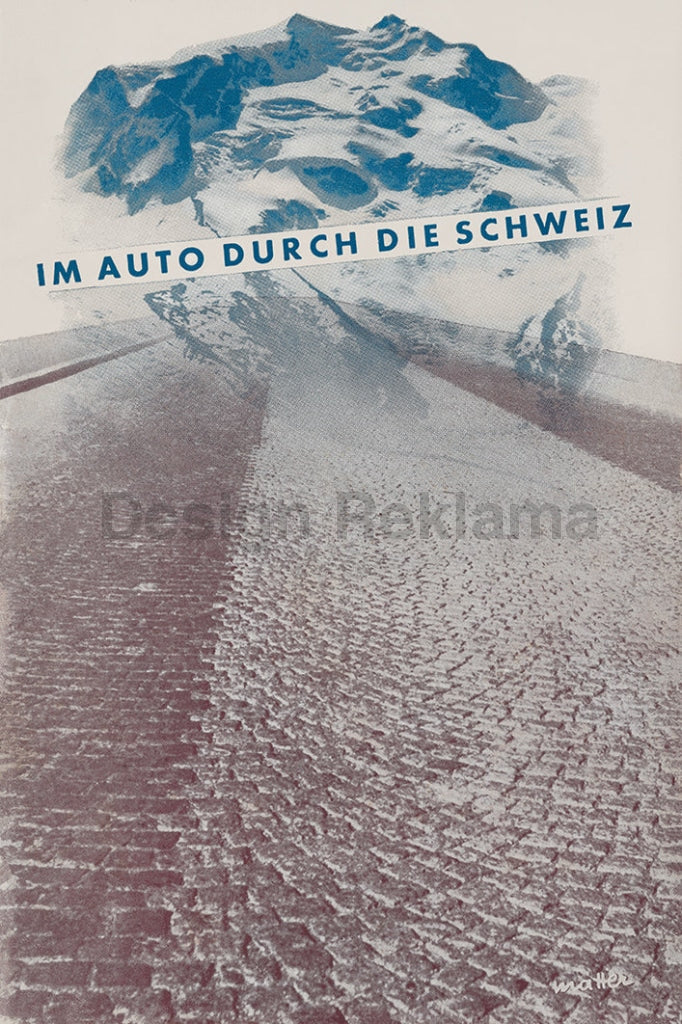The image features a monochromatic, out-of-focus illustration that blends elements of drawing and photography. Dominating the lower portion of the image is a reddish brick or cobblestone road, extending towards a seemingly endless horizon. The road is detailed with subtle shading and bounded by indistinct borders. In the upper part of the illustration, there are translucent, bluish-white mountains, evoking a snowy landscape. Faded letters spell out "DESIAN RAKLAMA," and beneath the mountainous scene, a banner reads “I'm Otto Dirk Deischweiss” or “I'm autodurch die Schweiz.” The overall composition of the image gives it a picturesque, yet abstract and enigmatic quality, leaving much open to interpretation.